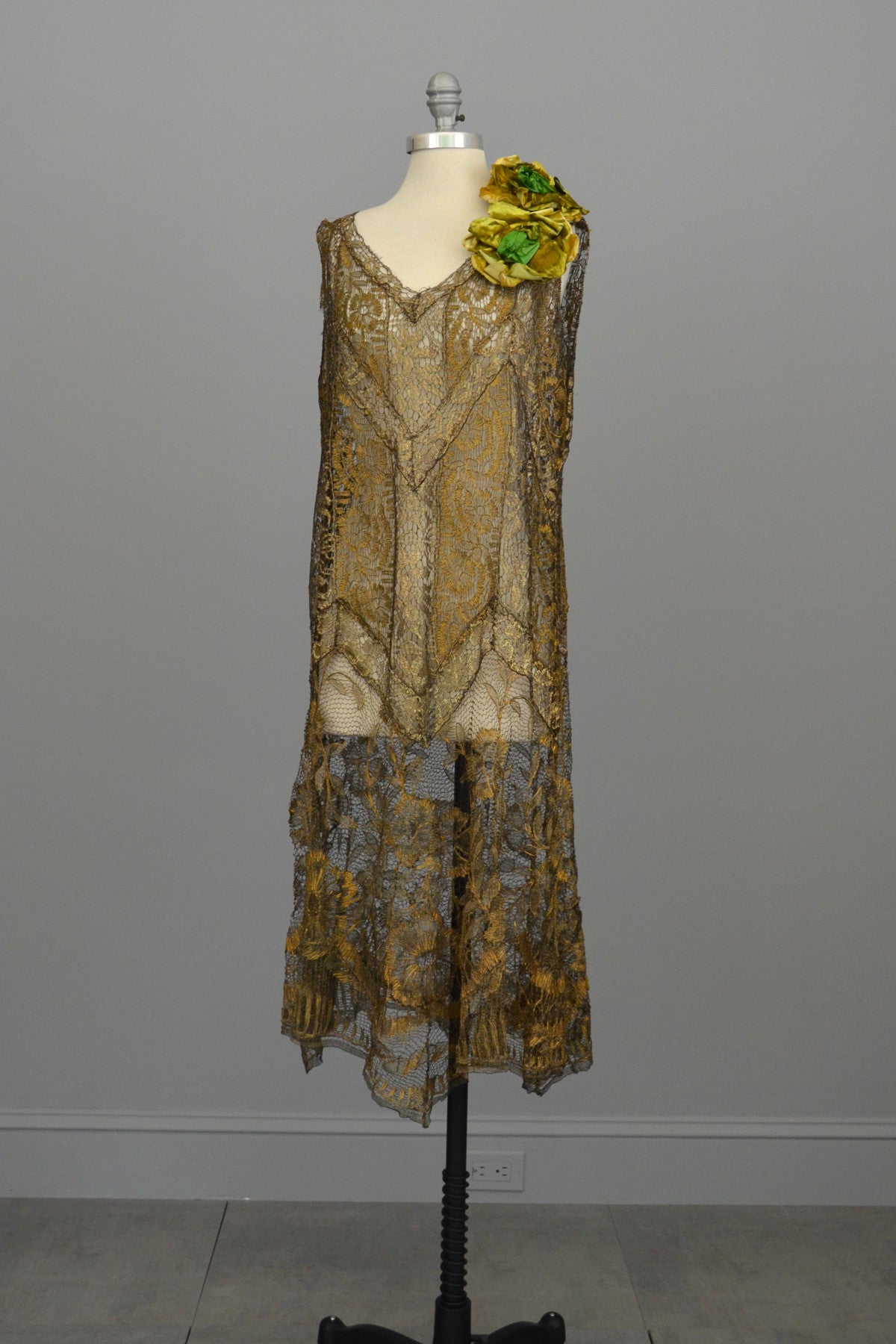This photograph features a vintage 1920s flapper dress displayed on a headless partial mannequin, which is sitting on a black stand against a grey background with a grey tiled floor and a visible wall socket. The dress, made from a very transparent sheer material with a muted golden brown or nicotine-stained hue, exhibits a delicate, lace-like quality. Intricate floral designs swirl throughout the fabric, segmented by lined sections, adding to the dress's ornate detail. Most prominently, the left shoulder is embellished with two large, worn yellow fabric flowers with grey centers. The overall aesthetic of the dress and display hints that it might be a product photograph intended for online platforms like Etsy or eBay.